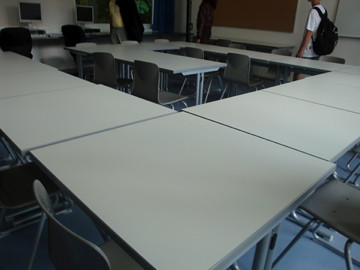A color photograph captures a school classroom with a distinct desk arrangement resembling a swirl or maze. The desks are simple white squares, each paired with a gray plastic chair featuring silver or gray metal railings. The desk formation starts from the top left, spirals toward the center, and ends in the bottom middle. The flooring is a lightly colored blue linoleum.

In the classroom, several objects are visible on the walls, including a large cork board in the top right corner and a whiteboard adjacent to it. In the upper left part of the image, two computer monitors are stationed on a separate desk. The walls of the room are white.

There are three figures in the background. The central figure is a young man wearing a white t-shirt and carrying a thick black backpack. To his left, there is possibly a teacher dressed in a yellow shirt and tan slacks, with a black jacket draped over his shoulder. The third person, situated centrally, appears to be wearing dark attire, possibly a jacket or a shirt. The classroom environment appears busy, with various items filling the corners and walls.